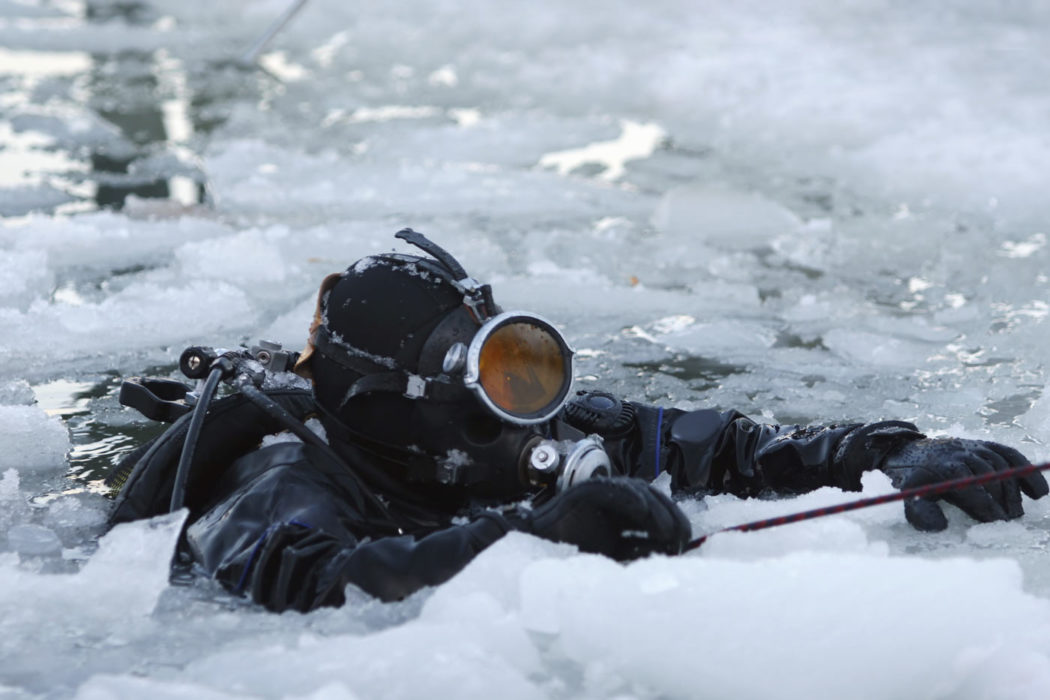The image depicts a scuba diver in an icy environment, likely a frozen lake, either in the process of entering or exiting the water. The surroundings feature numerous sections of broken ice revealing frigid water beneath. The diver, positioned slightly to the left and viewed from a top-down perspective, is dressed in a black diving suit, fully equipped with an oxygen tank and a face mask with a central, single glass piece. Tubes extend from the diver's mouth to the tank on his back. Additionally, the diver is holding a string or line that appears to be red or burgundy in color, extending to the right side of the image. The scene is captured during daylight, highlighting the contrast between the diver's dark gear and the icy surface.